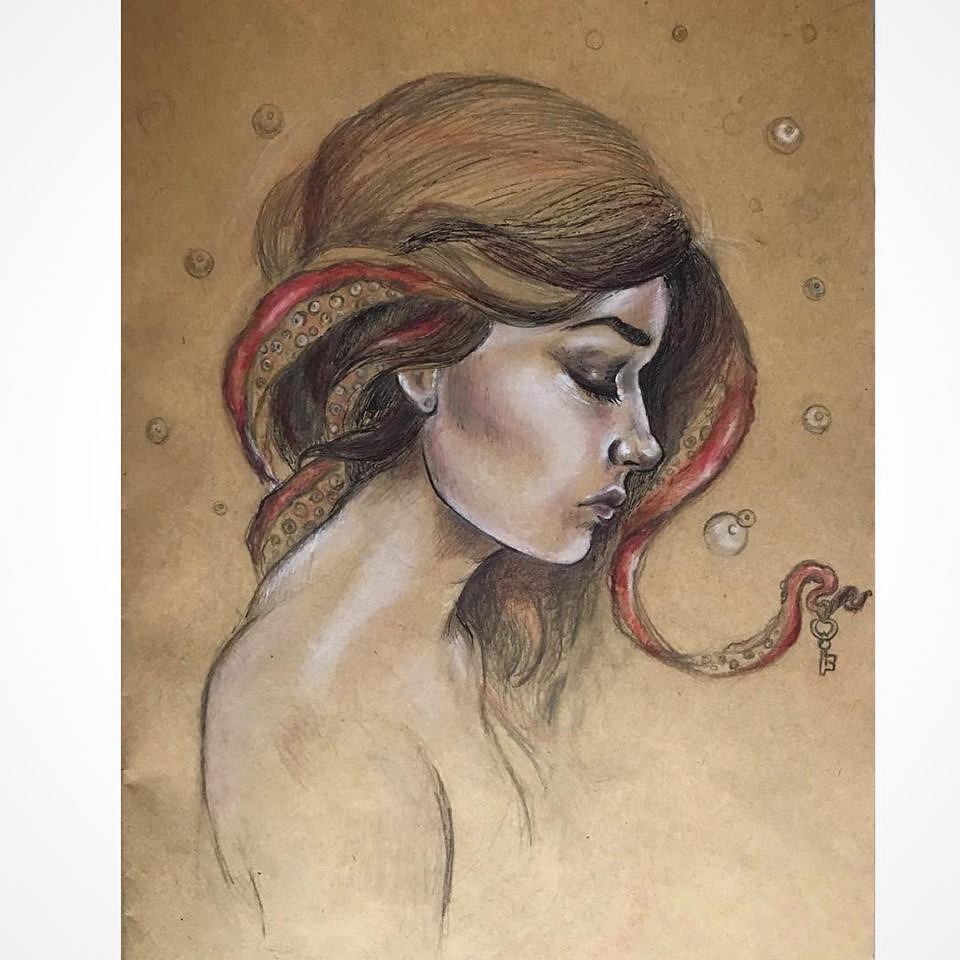The artwork depicts a detailed pencil drawing of a young woman in profile, emphasizing her serene and slightly melancholic expression. Her eyes are closed, and she exudes an air of quiet sadness. The image captures her from the shoulders up, revealing golden brown hair with a hint of red. Intriguingly, her hair is interwoven with octopus-like tentacles, some of which are red and adorned with small jewels or suction cup-like designs. One prominent tentacle extends outward, elegantly holding a skeleton key at its tip. The background features a rich brown hue, accentuated by delicate, bubble-like or pearl elements that further enhance the ethereal and surreal quality of the image.